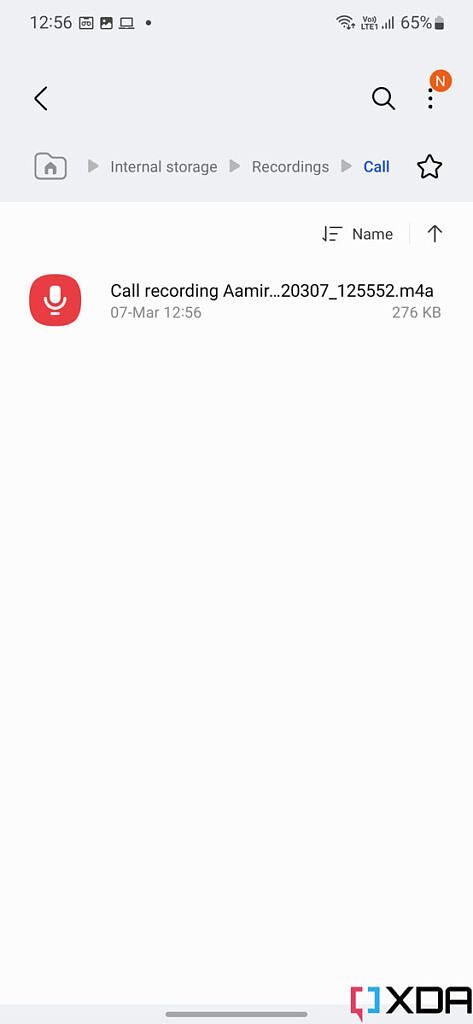This screenshot, captured from a smartphone, showcases various system icons and file details. At the top of the image, the status bar displays key information: the time reads 12:56, full Wi-Fi signal strength is indicated, and VOX LTE 1 shows robust four-bar phone coverage. The battery icon indicates a 65% charge. 

Beneath these icons, a file navigation path is visible: a folder icon containing a house symbol, pointing to "internal storage," then "recordings," and finally "call." Adjacent to this path is a star icon. Below these elements, a prominent red square with rounded corners houses a white microphone icon, denoting the presence of an audio file. The file is named "Call Recording AAMIR...20307_125552.M4A," created on March 7th at 12:56 PM, with a file size of 276KB.

In the bottom right corner, there's a text bubble icon, split in half with red and blue colors, labeled with "XDA" in bold black capital letters.